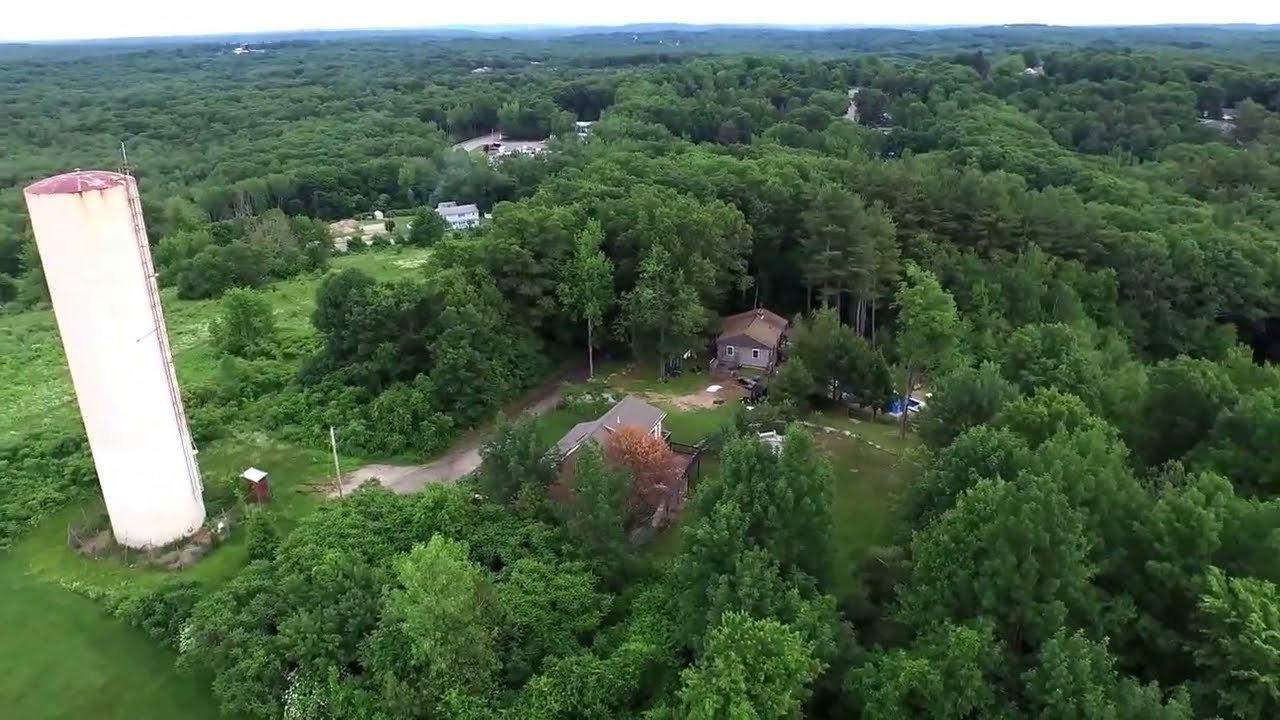The aerial view photograph captures a vast, densely forested area with vibrant, bushy green trees surrounding a small clearing at the center. Nestled in this clearing are a few gray-colored houses, one with a brown roof and another with a gray roof, linked by dirt paths winding through the forest. To the left of this central area, there is a prominent tall, white silo or cylindrical building set in another clearing devoid of trees, accompanied by a small rectangular structure which might be a utility building. The forest stretches extensively in the background with a few breaks in the canopy revealing scattered small, white buildings partially hidden among the trees. The scene is viewed from a significant height, giving the landscape an almost moss-like appearance due to the depth and lushness of the green foliage. The overall composition forms a distinctive pattern with the houses and structures interspersed within the natural expanse of the forest.